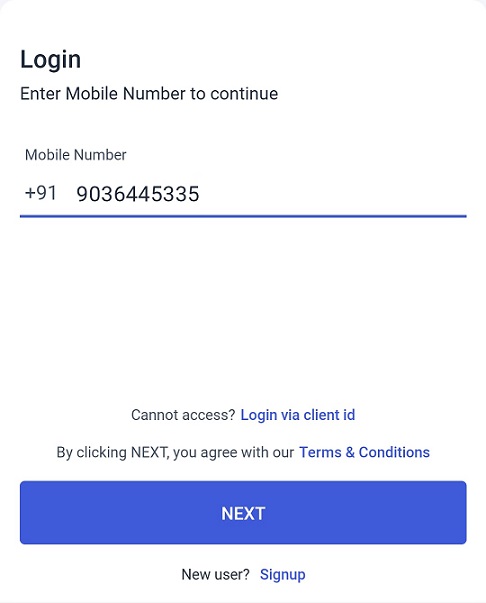This cropped screenshot showcases a portion of a website with a clean, white background. At the top left corner, a light gray triangle is prominently visible. To the right of this triangle, bolded black text reads "Login," with a corresponding smaller line of black text below it stating, "Enter mobile number to continue." 

Beneath this instruction, another line break reveals slightly indented, small black text labeled "Mobile Number." Following another line break, larger black numerals display the format "+91 9036445335," which is underlined in thick medium blue. 

A significant area of negative space separates this section from centered light gray text that reads, "Cannot access," which is paired with blue text to its right stating, "login via client ID." Note that "ID" is written in lowercase.

Further down, centered light gray text informs, "BY CLICKING NEXT, YOU AGREE WITH OUR," followed by blue text titled, "terms and conditions." Below this message, there is a purplish-blue button spanning almost the page's full width, featuring all-caps white text in its center that reads "NEXT." 

At the bottom, centered black text states, "New user," followed by blue text to the right saying, "sign up," written as one word. The page concludes with a thin light gray line just beneath this final line of text. Another light gray triangle is situated in the top right corner of the page, mirroring the one on the left. Additionally, there is a minor area of negative space at the top right, balancing the design elements of the page.